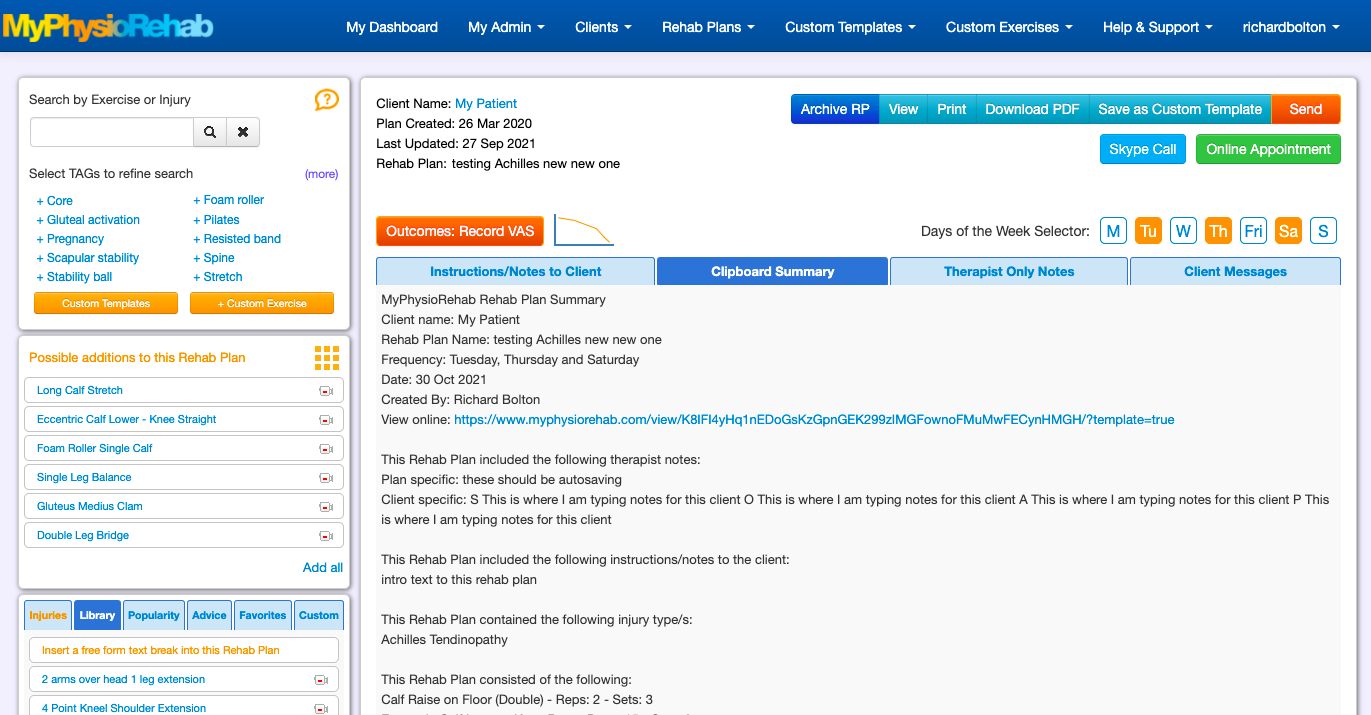Screenshot Description:

The image is a screenshot of the user interface for a program called "My Physio Rehab." The program's name is prominently displayed in the top left corner of the menu bar against a blue background, with "My Physio" rendered in a gradient of orange and yellow, and "Rehab" in blue. The remainder of the menu items are listed in white text and include: My Dashboard, My Admin, Clients, Rehab Plans, Custom Templates, Custom Exercises, Help and Support, and Richard Bolton. Each menu item, except for My Dashboard, has a small drop-down menu icon next to it, indicating the presence of additional sub-options.

On the left-hand side of the interface, there is a column containing three sections dedicated to search and filter options. These options allow users to search by various criteria such as exercise type or injury. Examples of exercise types that can be searched include foam roller, Pilates, resistive band, pregnancy, and stability ball. Users also have the ability to choose custom templates or custom exercises and add different exercises to a rehab plan.

On the right-hand side, the interface displays a client profile, presumably with relevant information and details about the client’s rehabilitation journey. Additional options accessible via the interface include writing instructions or notes to the client, accessing a clipboard summary, viewing therapist-only notes, or reading client messages. 

The overall layout is designed to provide comprehensive functionalities for managing and customizing rehabilitation plans within the "My Physio Rehab" program.